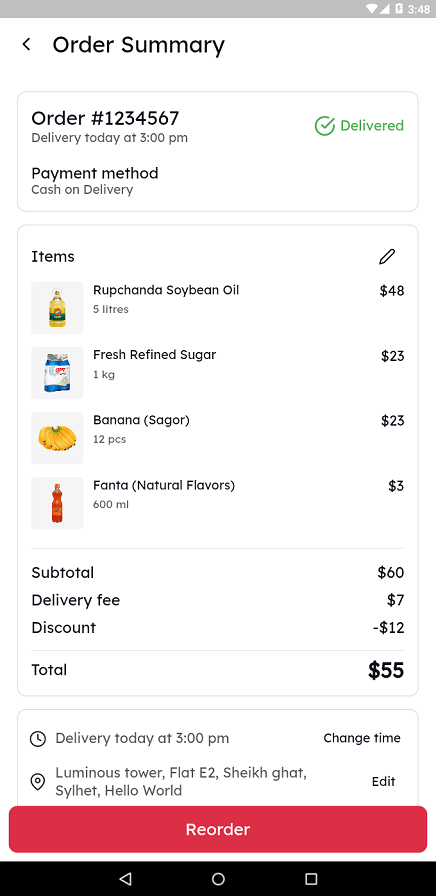The image is a cell phone screenshot with a clean white background. At the top, there is a gray rectangle stretching across the screen, housing all the cell phone status icons in white on the right side. Directly below, aligned to the left, a small black arrow pointing to the left resembles a sideways V. Adjacent to the arrow, in large, bold black letters, is the title "Order Summary."

Beneath the title is a light gray outlined rectangle containing the order details. Positioned at the top-left corner, it displays the order number. Just below this, in smaller gray text, it reads "Delivery today at 3 p.m." On the right side of the rectangle, there is an outlined green oval with a checkmark inside it. Beside this green oval, the word "Delivered" is written in green.

Two lines down, on the left, is the heading "Payment Method," followed by the phrase "Cash on Delivery" just below it. Further down is another light gray outlined rectangle listing the contents of the order. The top-left corner inside this rectangle labels the section "Items," and to its right is a pencil icon allowing for edits. Each ordered item is presented with a small square image of the product on the left, the item’s name to the immediate right, and the price aligned to the far right edge, marked with a dollar sign.

Following the items list, there are sections for "Subtotal," "Delivery Fee," "Discount," and the final "Total" with their respective values. Additional information regarding the delivery time and destination is also displayed. At the very bottom of the screenshot, there is a prominent horizontal red rectangle labeled "Reorder" with the text written in white.